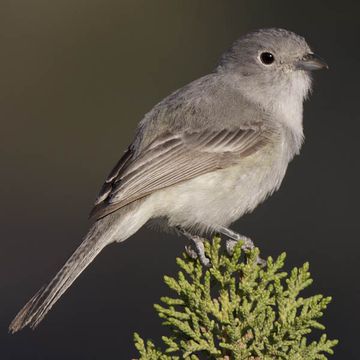The color photograph features a small bird, likely a sparrow or finch, perched on a green branch that resembles a pine or evergreen bush. The bird, with its rounded body and gray feathered coat, stands slightly off-center towards the right, presenting a full side profile. It has a small black beak, a rounded eye, and its tail angled towards the bottom left. The background is a solid dark gray with varying shades providing a muted contrast to the bird's light gray chest and slightly darker gray upper body. The green branches extend from the bottom right, while the bird's claws grip firmly, enhancing the natural setting of the image.